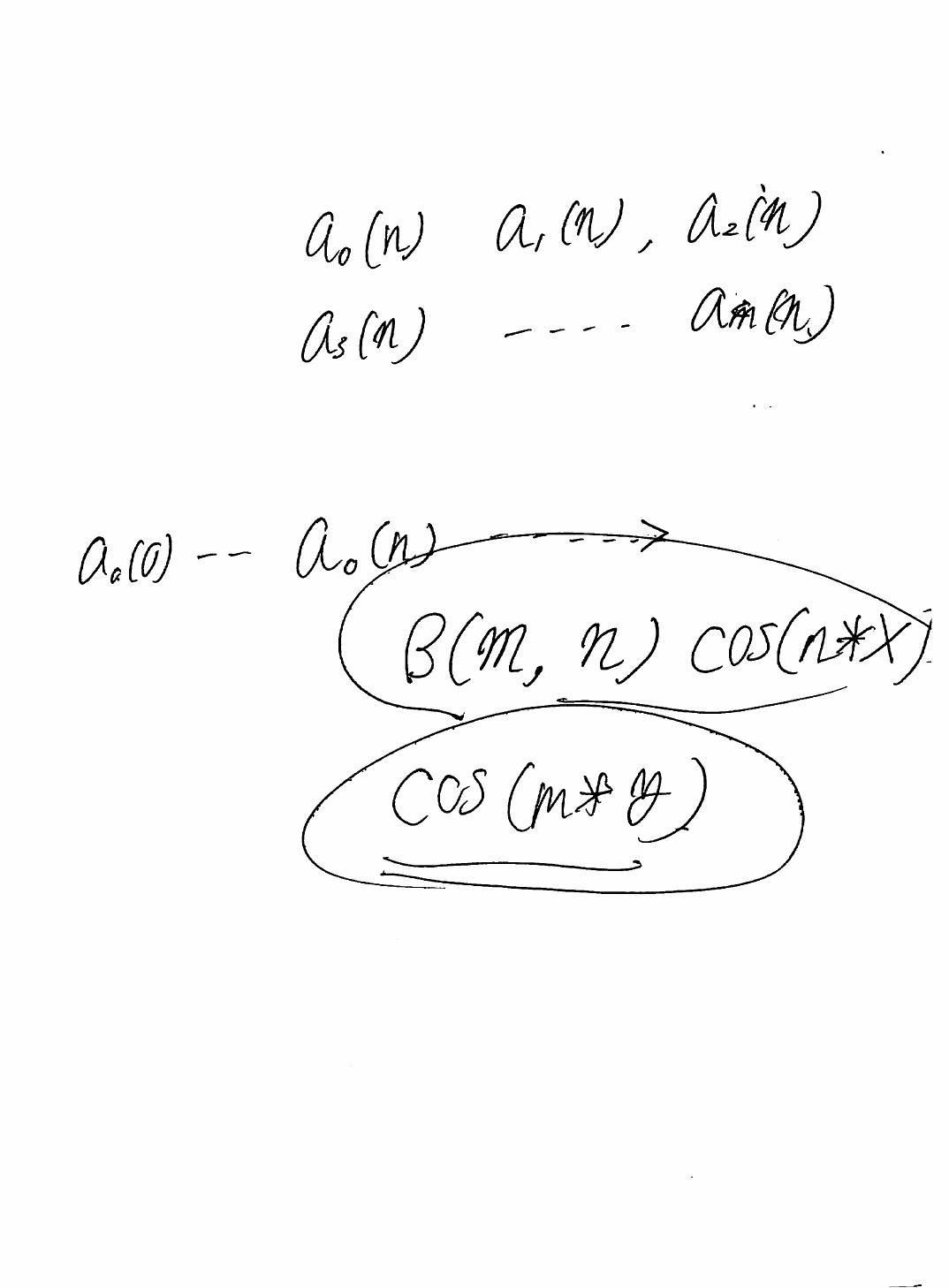This photograph showcases a meticulously handwritten set of mathematical or chemical formulas on a sheet of white paper. The notes are inscribed in black pen with remarkably uniform and legible handwriting, indicating careful attention to detail. At the top of the page, there are symbols followed by the letter "N" in brackets, repeated three times across the line. Below this line, the same symbol with a zero in brackets appears, followed by two hyphens, the symbol again, the letter "N," and then an ellipsis (dot dot dot) with an arrow pointing to the right.

Further down the page, a formula has been neatly circled and beneath it, another formula has been both circled and underlined. The first formula reads "B(M, N) COS(N * X)," and the second one below it is "COS(MXY)," both circled and the latter also underlined for emphasis. The careful arrangement and clarity of the formulas suggest a methodical approach, possibly indicating a set of steps or processes central to the written content.